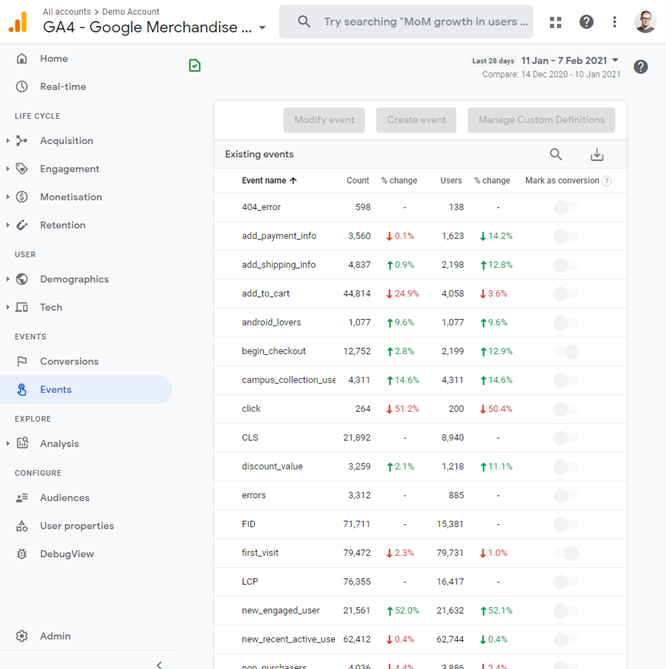This screenshot depicts a Google analytics dashboard, offering detailed insights and statistics. At the very top, a white header bar houses essential navigation and utility features. The top left corner features text indicating "All Accounts" with an arrow pointing to "Demo Account". Just below this, there's the label "GA4-Google Merchandise" accompanied by a logo, likely representing the Google Analytics program in use.

Moving to the right side of the header, a search bar allows users to perform queries within the dashboard. Adjacent icons include a grid of four squares for additional options, a question mark inside a circle for help, and an ellipsis for more settings. The header concludes with a small portrait image of a white man wearing glasses, presumably representing the current user logged into the account.

Beneath the header, the main webpage is dominated by an event log detailing various activities. Central to the screen is a window displaying existing events, complete with event names, counts, change percentages, and user change percentages. Users also have the option to mark these events as conversions. The displayed events span a range of actions such as "404 error" and "add_payment_info," all accompanied by quantitative data.

On the left-hand side of the screen, a vertical sidebar provides navigation through various sections of the dashboard. Tabs include "Home," "Real Time," "Life Cycle," "User," "Events," "Explore," and "Configure," allowing users to seamlessly cycle through different parts of the analytics tool.

In summary, this comprehensive analytics page offers an array of data points and navigation tools, catering to users seeking in-depth information about their digital activities within Google's platform.